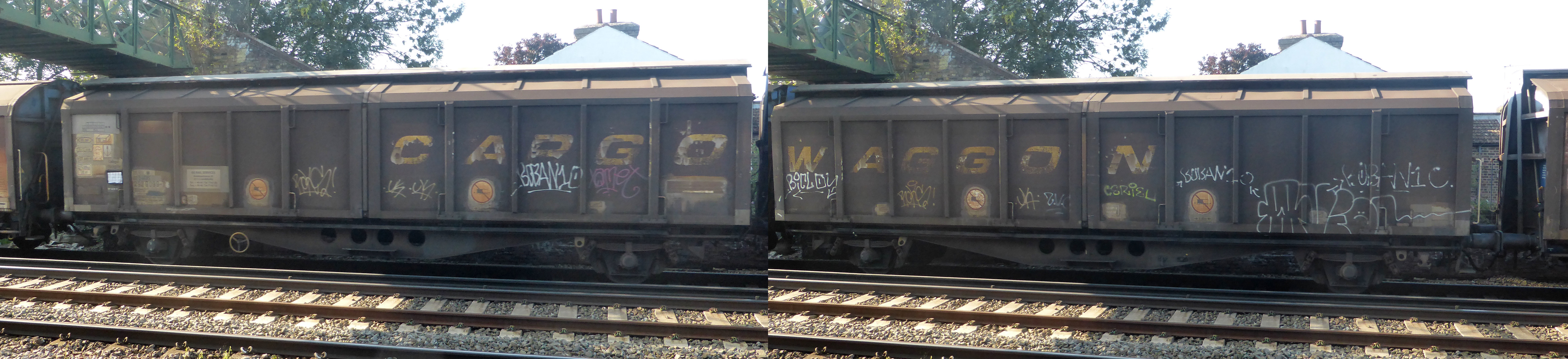These side-by-side photographs show two similar cargo train cars positioned on wooden and metal train tracks, amidst loose pebble-like gravel. The background reveals the top roof of a building, a green bridge on the top left, and trees with a bright white sky in the upper right. The train car on the left is dark brown with faded yellow letters spelling "CARGO," and features graffiti in yellow, white, and a bit of pink. The right photo showcases an identical style train car, with the yellow text "WAGON" and similar graffiti beneath it. Both cars are rusty and enclosed, indicating the contents are protected. Despite their graffiti being covered partially with white paint, the overall decrepit charm is prominently visible.